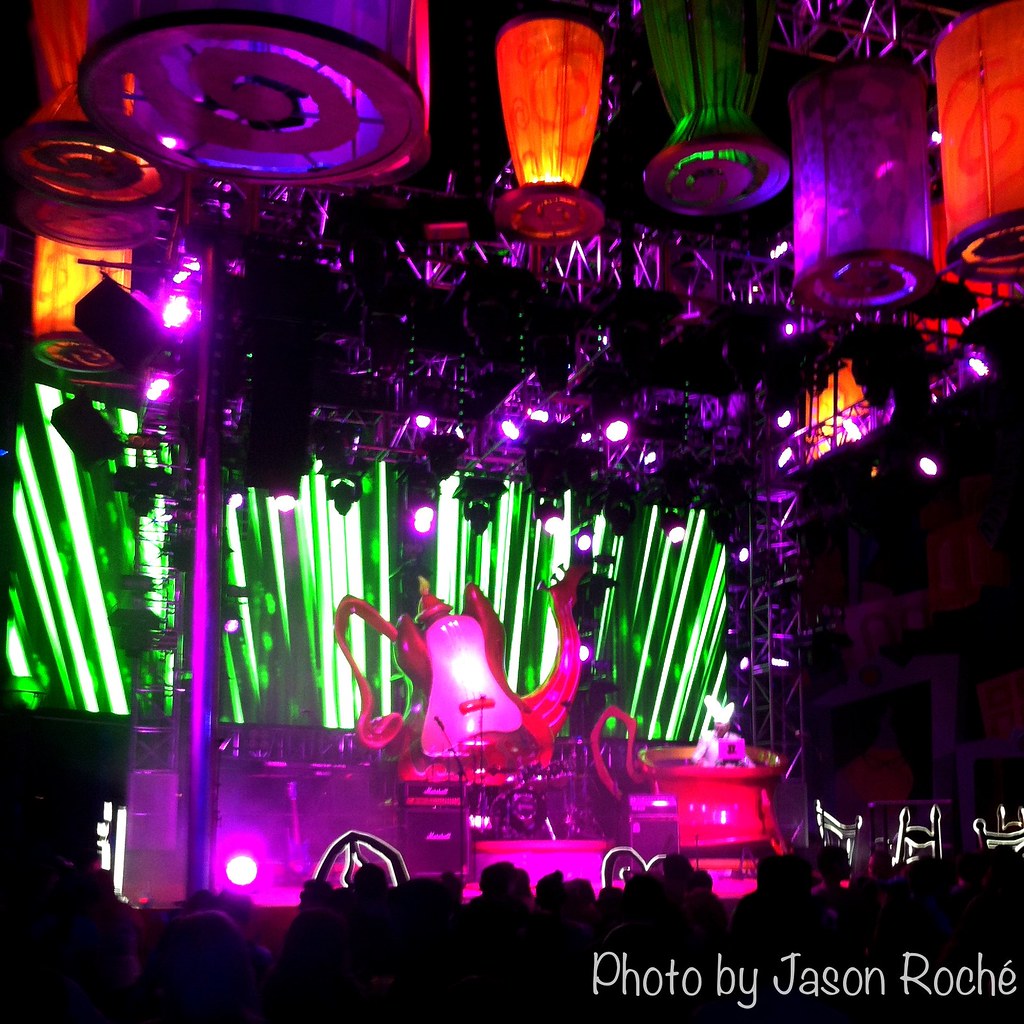This vibrant nighttime photo, taken by Jason Roche, captures the lively atmosphere of an interior music club illuminated by multi-colored neon lights. Dominating the scene are red, green, purple, pink, and orange skylights that hang from the ceiling, bathing the space in a radiant glow. At the top of the image, iron framework supports additional lights, enhancing the vivid ambiance.

The stage backdrop features striking green vertical stripes, resembling illuminated bars. In the foreground, an intriguing teapot-shaped sculpture catches the eye; its spout adorned with three guitar adjustment knobs, the body mimicking a guitar's form, and a handle on its left side. Surrounding the stage are various amplifiers and other musical equipment, suggesting preparation for a performance.

The photograph, although slightly blurred, clearly depicts a bustling crowd silhouetted against the stage, with some audience members standing and a few chairs visible on the right side. Despite the lack of identifying information about the event, the image exudes a colorful and energetic nightlife scene.